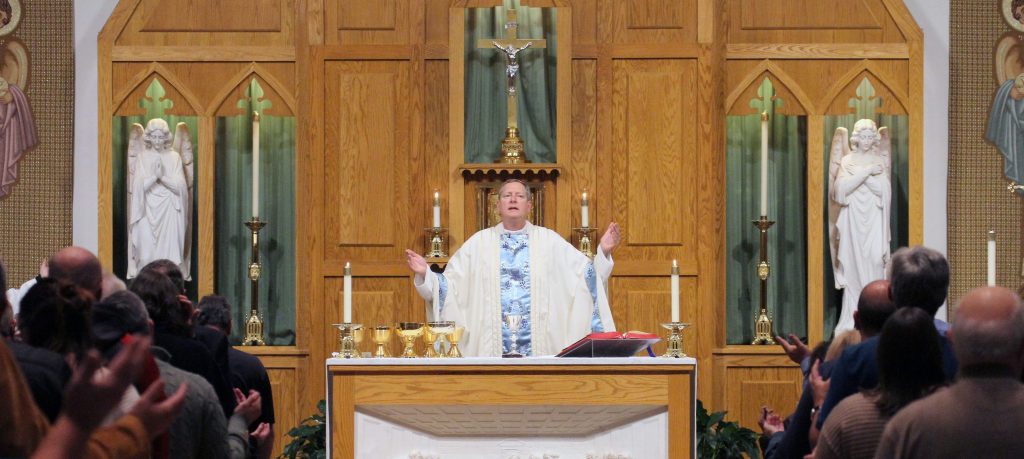This photograph captures a solemn moment during a Mass inside a Catholic Church. In the focal point of the image is a white male priest, dressed in white robes adorned with light blue satin detailing, standing behind the altar with his hands raised in prayer. Surrounding him, the congregation fills the pews with their hands similarly upraised.

The altar is adorned with an array of ceremonial items: several golden chalices on the left side, an open Bible on a stand with red-edged pages on the right, and two tall white taper candles in ornate candlesticks. Behind the priest, a wooden backdrop features a prominent crucifix with Jesus hanging above the priest's head, flanked by two marble statues of angels. One angel stands with hands together in prayer, while the other has arms crossed over her chest. The scene is enriched with the detail of golden pale oak wooden moldings, adding to the sacred ambiance of the church.